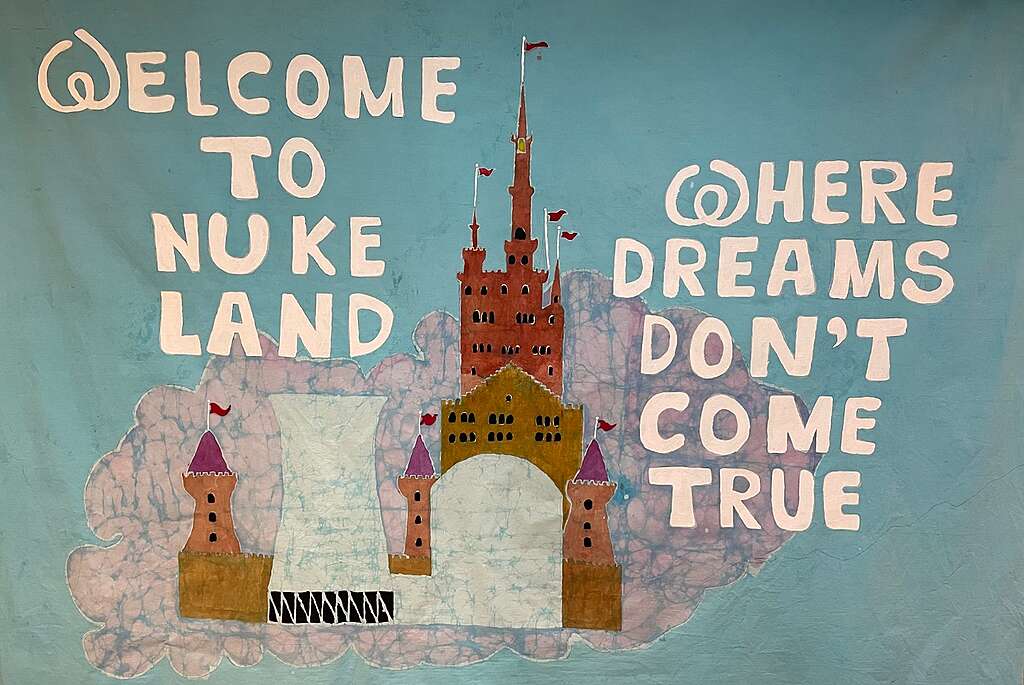The illustration depicts a surreal, artistic representation featuring a distressed cloud-like form against a subtle white and blue background resembling a wall. The cloud appears weathered and fractured with blue cracks, evoking a sense of decay and disintegration. Embedded within the cloud is a detailed depiction of a medieval fantasy castle, complete with flags, turrets, and towers. Uniquely, one section of the castle transitions into the exhaust stack of a nuclear power plant, blending the whimsical with the industrial. Overlaying the scene, in stark white text, is the unsettling phrase: "Welcome to Nuke Land, where dreams don't come true."